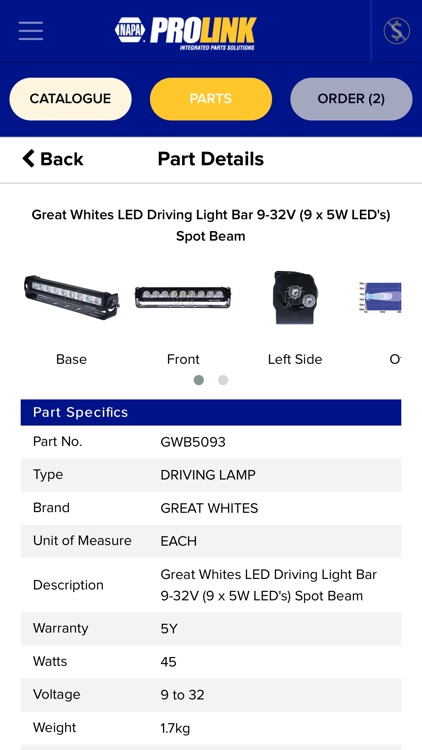This image features the NAPPA ProLink Automatic Parts Distributors interface. The topmost section displays the "Automated Parts Distributors" text within a blue bar. Below this bar, a secondary blue bar contains three distinct buttons. 

Starting from the left, the first button is light tan with black, all-capital letters, labeled "CATALOG." The middle button stands out in yellow with white, all-capital letters, labeled "PARTS." The third button on the right is gray with a black, all-capital-lettered label "ORDER," accompanied by the number two in parentheses, indicating the order quantity.

Beneath these buttons is a detailed Part Details section. It lists four specific items: "Base," "Front," "Left Side," and a partially visible item due to cutoff. This section provides a structured and organized view of part specifics, aiding in efficient inventory management and order processing.